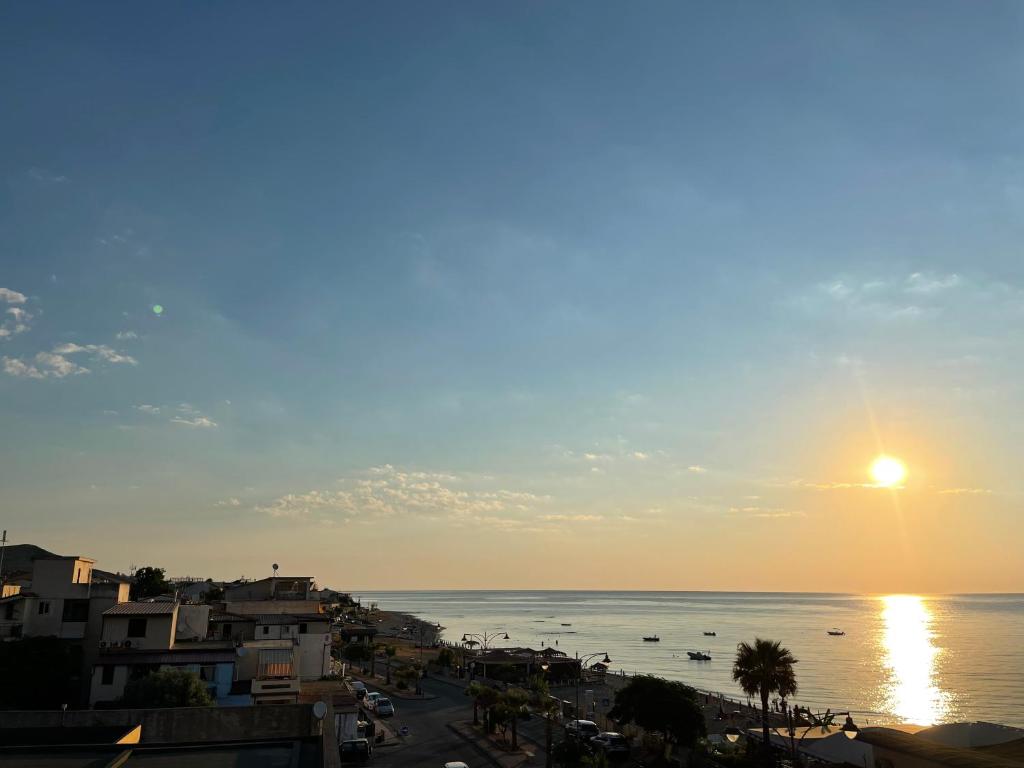This is a high-angle shot capturing a picturesque coastal city at sunset, likely taken from a balcony or higher ground. The horizon is situated in the lower third of the image. We look out over a waterfront town nestled beside a tranquil ocean, with the beach stretching below us on the right side of the photo. The cityscape on the left is peppered with a mix of apartment buildings and cars parked along the streets, and a few palm trees adding a tropical touch to the scene, reminiscent of coastal Portugal. 

The ocean, tinged with bluish-gray tones, reflects the setting sun's jagged strip of golden light, which dances across the water's ripples. The sky above transitions from hazy orange near the horizon to a clearer blue further up, punctuated by a light scattering of grayish-white clouds. Down on the shoreline, a boardwalk can be seen bustling with people, flanked by beachside restaurants and small personal boats dotting the water. The buildings, beach, and boardwalk below are bathed in the soft, backlit glow of twilight, casting long shadows and evoking a serene, almost magical, ambiance.